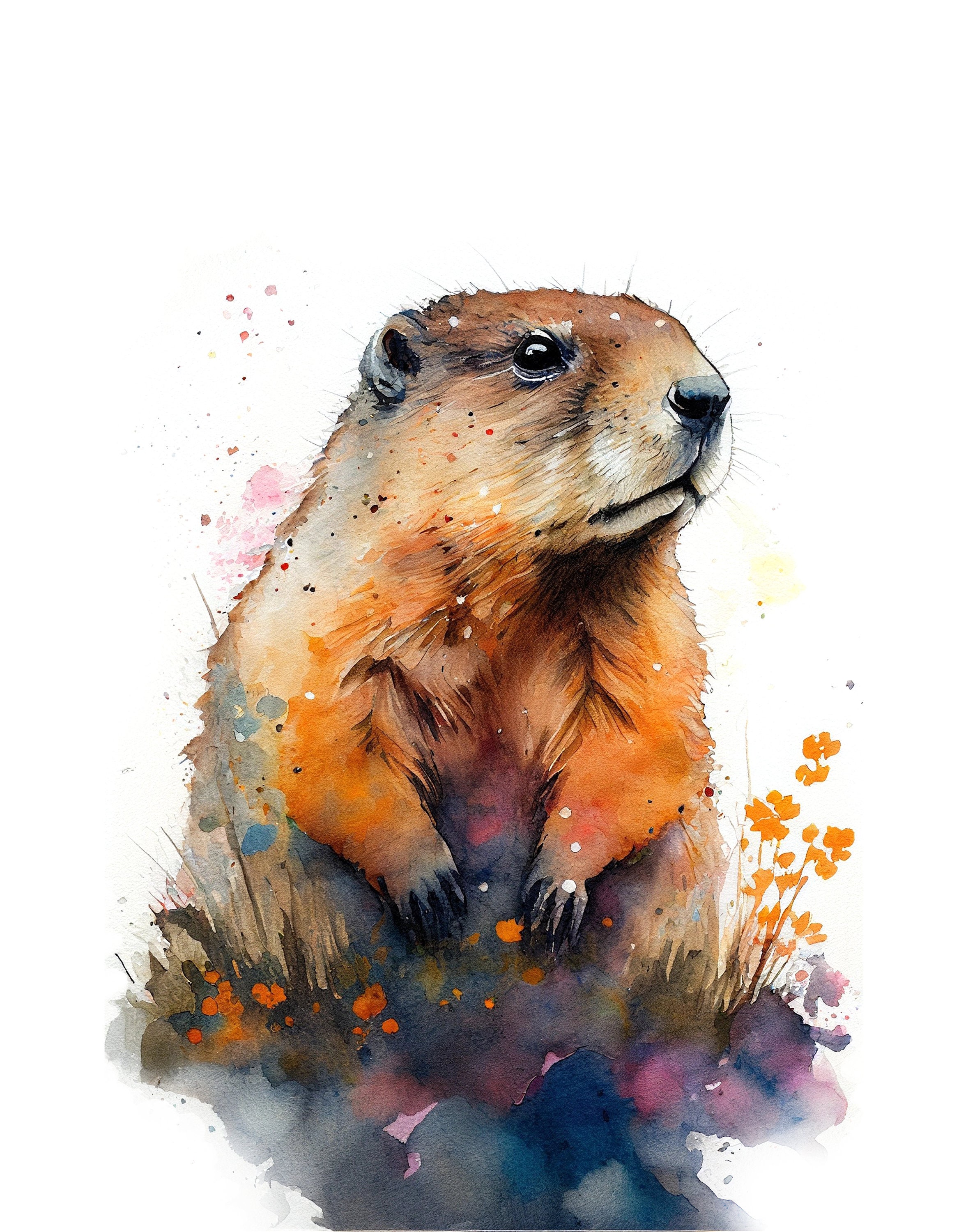This detailed, watercolor painting on a white sublimated background features an adorable groundhog standing upright on its haunches. The groundhog is depicted from its midsection upward, with its bottom half obscured by various colorful elements. The animal's fur exhibits a rich gradient: its face is a soft brown that fades to a light tan under the eyes and a white muzzle adorned with black whiskers. Small, rounded, furred ears sit close to its skull, while its expressive wide eyes, small nose, and subtly chinned mouth add to its charm. 

The groundhog's forepaws, draped elegantly in front of its body, are a distinctive reddish-brown. It appears to be looking to the right, showcasing a side view of its right eye, ear, and closed mouth. The area around its body is lively with watercolor foliage and flowers; green leaves and bright orange-yellow petals mingle with gray and dark rocks at the base. Pink, tan, and gray splatters artistically decorate the background, adding a whimsical touch to the composition. The lower part of the groundhog's body blends seamlessly into this vibrant flora, with hints of purple, blue, and green rocks enhancing the scene's richness. This exquisite, text-free artwork vividly captures the charming essence of the groundhog amidst a colorful, nature-inspired setting.